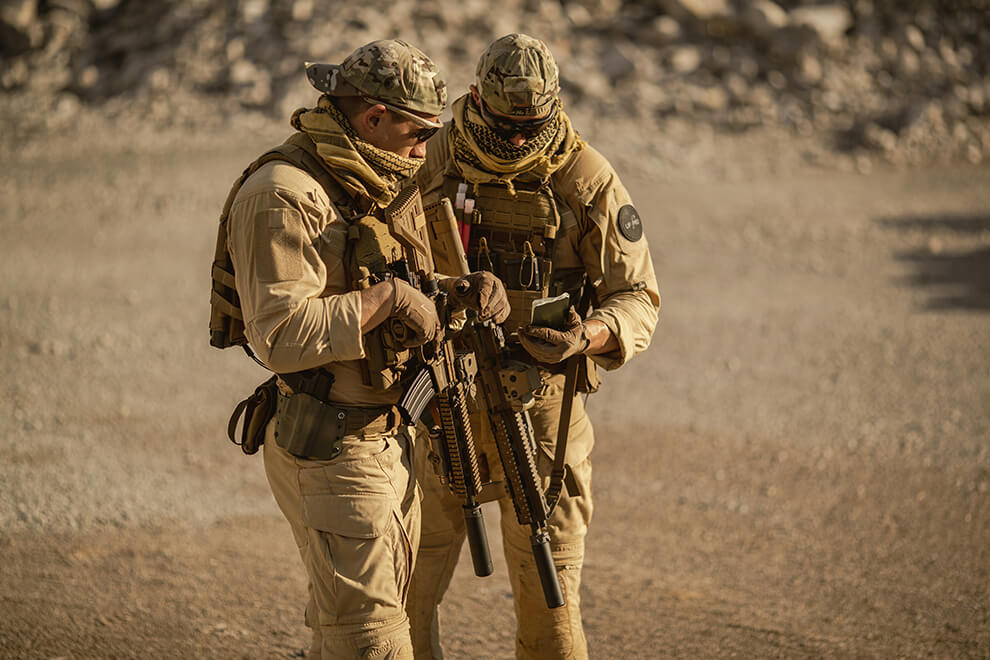This photograph features two soldiers standing closely together in a desert environment with a flat, tan dirt ground. Above, the shadow reflections of tree branches can be faintly seen. Both soldiers are dressed in full light tan military uniforms, complete with long-sleeved shirts, cargo pants, and tan gloves. They each wear a camouflage baseball cap backwards and have black sunglasses shielding their eyes. Their faces are partially covered with scarves featuring a Middle Eastern brown and black checkered design, wrapped up to slightly below their noses.

The soldier on the left, sideways to the camera, sports a light tan uniform with noticeable details such as a scarf wrapped around his mouth and a yellowish hue. He has a utility belt strapped around his waist and carries a light tan rifle with a suppressor pointed downwards. His attention is fixed on an object—possibly a phone or a paper pad—held by the soldier on the right.

The soldier on the right wears a matching hat and scarf, with his left arm adorned with a patch on the sleeve. Like his companion, he also carries a tan rifle with a suppressor pointed down and has his gaze locked onto the electronic device or notebook in his left hand, which both are intently examining.